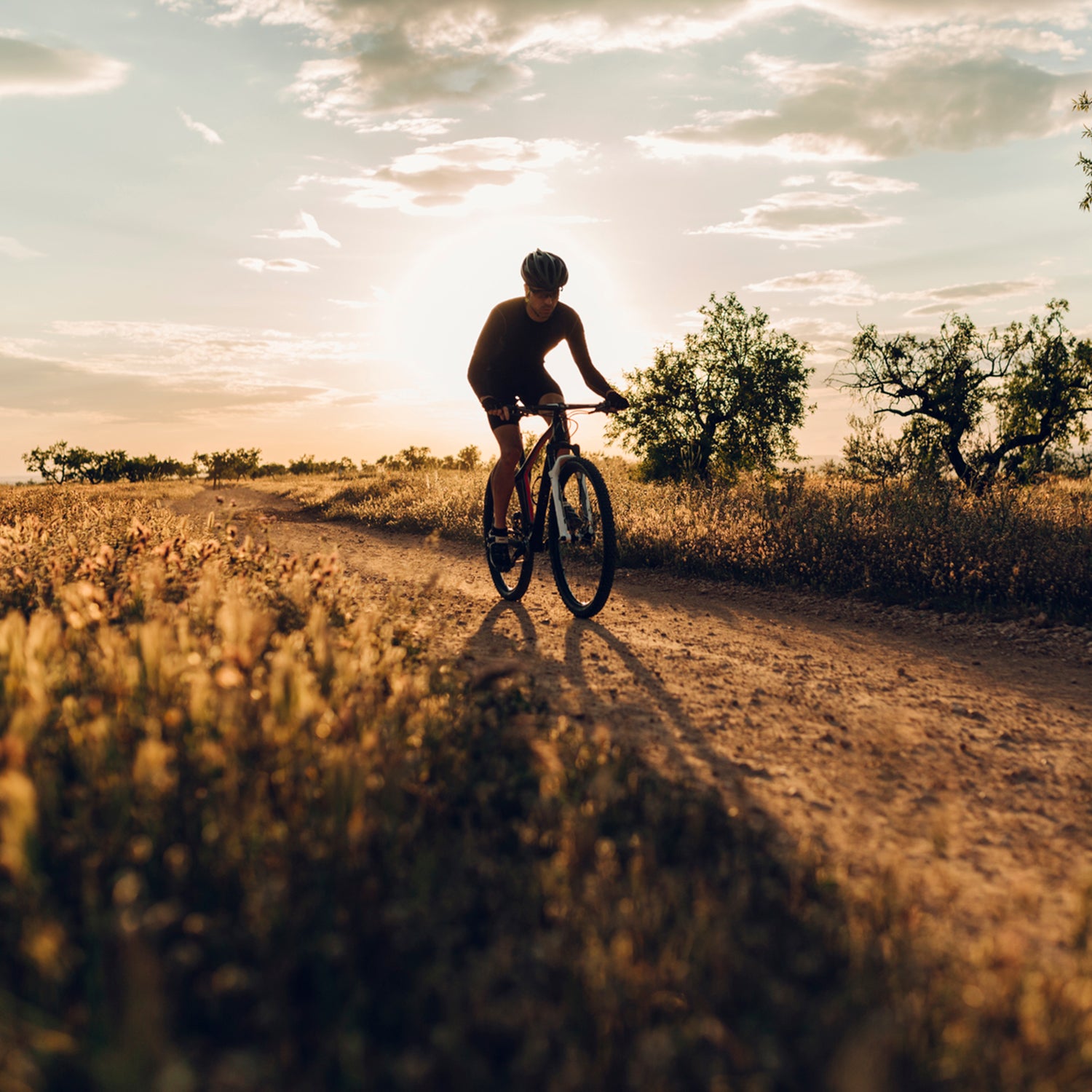The photograph captures a serene outdoor scene at either sunset or sunrise, with the sun positioned directly behind a man riding a bicycle, casting him into shadow. The central dirt path he traverses is flanked by high, dried brownish grass and warm brown tones dominate the image, giving it an overall golden hue. In the background, a pair of trees stand further back on the trail, accompanied by a few clouds scattered across the sunny sky, creating an idyllic, tranquil setting. The rider, who appears to be wearing a long-sleeved shirt, shorts, glasses, and a helmet, is indistinct due to the backlighting but is moving towards the camera, embodying the essence of a solitary, peaceful journey.